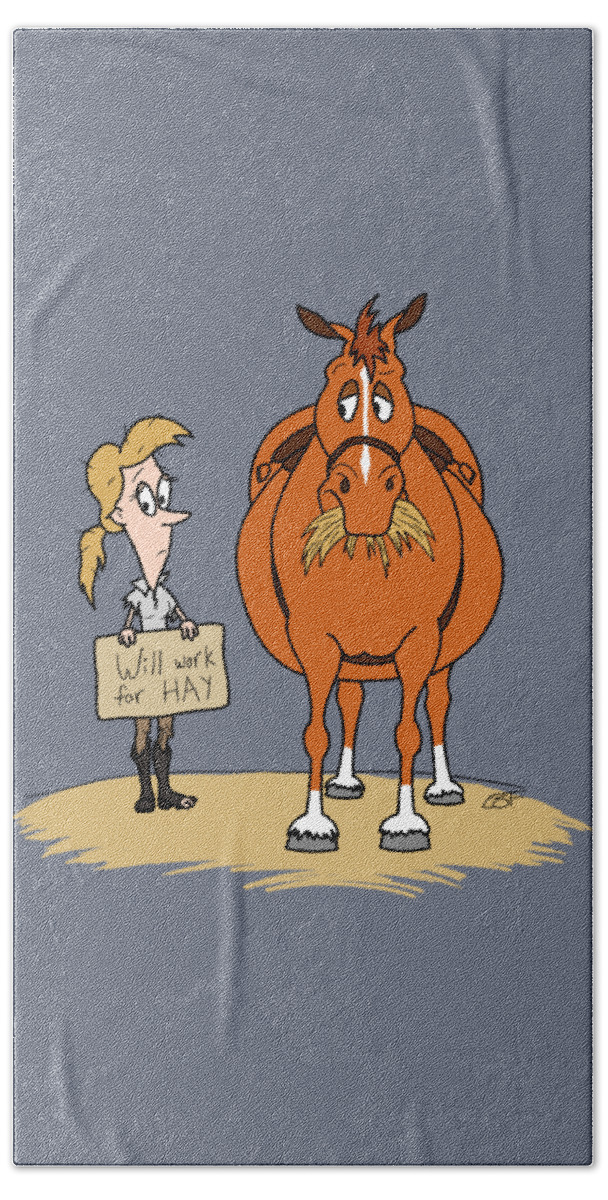This detailed photograph showcases a cartoon-like illustration, possibly rendered on a gray, textured fabric, akin to a t-shirt. The fabric's surface appears ridged, giving it a tactile depth. The image features a large, head-on view of an orange horse with a white stripe running down the middle of its head and a matching tuft of red hair. The horse, which has white hooves with gray bottoms and a dark brown saddle, is chewing on some hay. Its eyes are turned skeptically towards a woman standing to its left. The woman, who has straw-colored blonde hair tied in a ponytail, sports a blue short-sleeved shirt, brown leggings or pants, and high black boots. She holds a sign in her hands that reads, "Will work for hay." Both the horse and the woman are standing on a roughly sketched mound of brown hay, set against the textured gray backdrop.